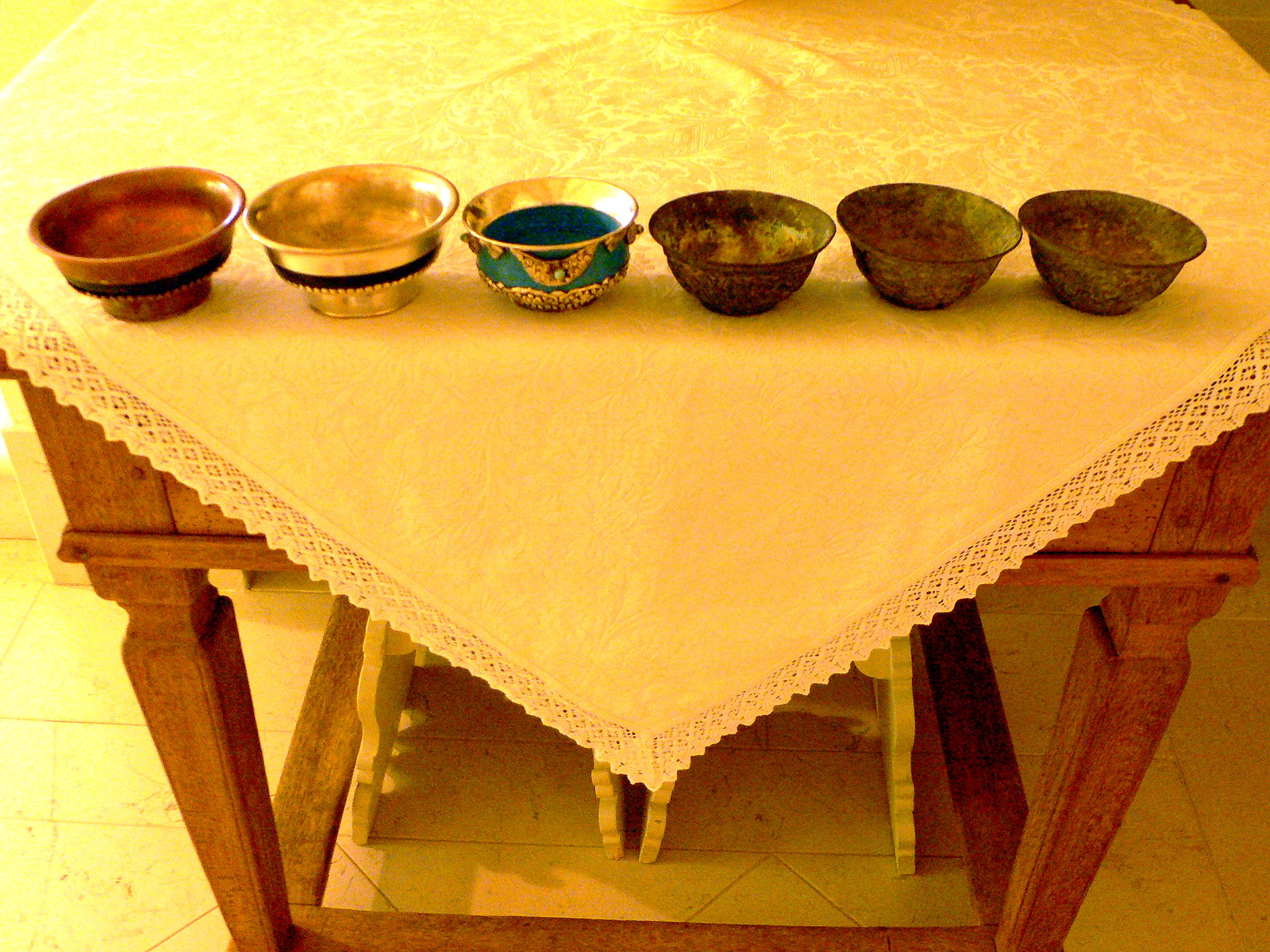This photograph captures a rustic wooden table adorned with a white linen tablecloth featuring delicate lace embroidery at the edges. The table, set against a pale-colored linoleum floor, is illuminated with a warm, yellowish light that gives the scene an antique feel. Positioned near the edge of the table in a neat row, the bowls are arranged in decreasing size from left to right. 

The largest bowl, on the far left, has a brass-like appearance, followed by a slightly smaller golden-colored bowl. Next in line is a smaller, rounded bowl with an ornate green enamel and gold decoration. The last three bowls are identical, made of dull pewter, showcasing a dark gray, hammered metal look complete with tarnish, enhancing their antique allure. This composition creates a harmonious blend of aged charm and subtle elegance.